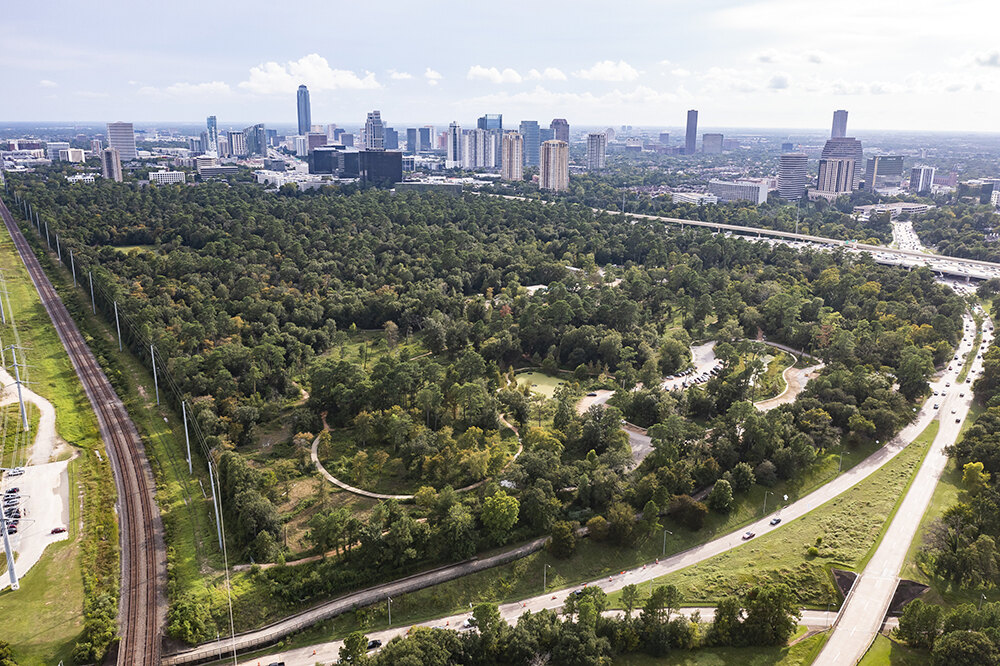This color photograph offers an expansive, aerial view of a large, rectangular-shaped park nestled within a bustling city. The image captures a scene brimming with verdant trees in full bloom, suggesting a summertime setting. In the foreground, a divided highway with visible cars runs along the edge of the park, while a large elevated highway can be seen further in the distance. On the far left side of the image, dual train tracks extend from the bottom left corner upward, flanked by power lines along the park's periphery.

The park itself is densely wooded with lush greenery and includes various jogging and biking paths weaving through its landscape. A man-made lake is situated within the park, potentially accompanied by recreational areas such as a skateboarding park. A parking area for cars is also visible on the right-hand side. The city's skyline looms in the background, characterized by numerous skyscrapers and apartment buildings, though the exact city remains unidentifiable and does not appear to be American. The daytime sky is hazy, possibly due to smog or air pollution, with grayish hues and some white clouds scattered throughout. The source of the image appears to be from a drone or a high-rise building adjacent to the park, providing a comprehensive overview of this urban oasis.